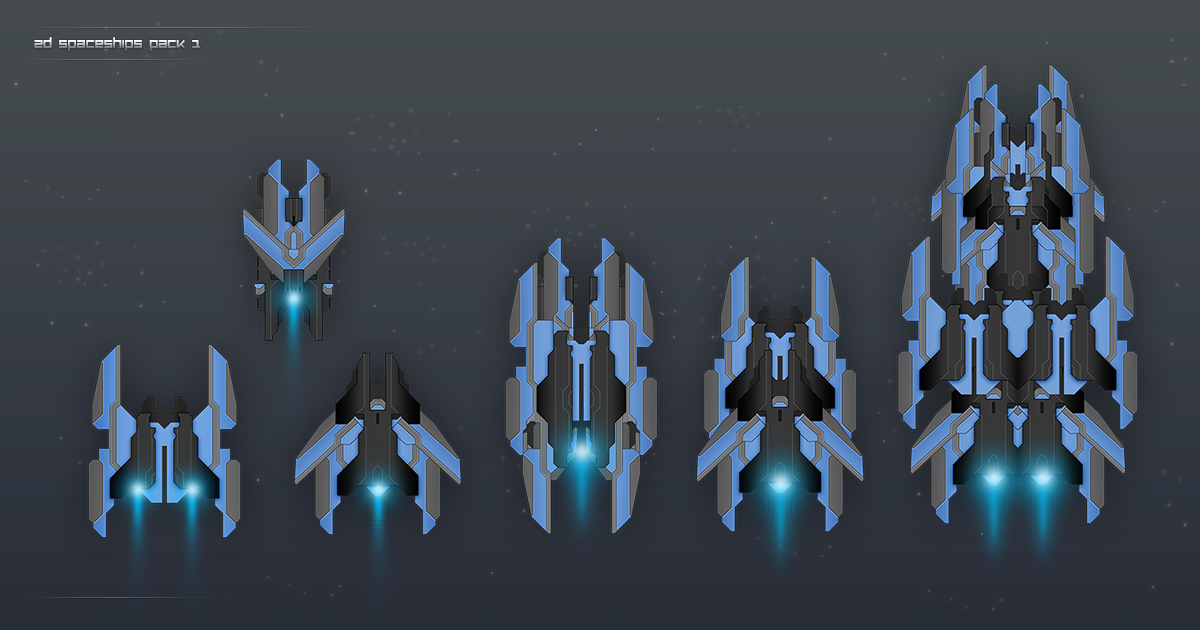This image appears to be a promotional or conceptual artwork for a video game asset titled "2D Spaceship Pack 3." Set against a dark gray background speckled with white dots resembling stars, the image showcases six distinct spaceships arranged neatly from left to right, in ascending order of size. The spaceships are designed in a cohesive aesthetic, with all of them featuring a consistent color palette of blue, gray, and black. They vary slightly in shape, with some exhibiting a triangular design while others resemble various forms, including bug-like shapes. Most of the spaceships have light blue propulsion beams at their rear, indicating their jet engines. The largest spaceship is notably four or five times the size of the smallest one, and the intermediate ships are of varied medium sizes. The caption "2D Spaceship Pack 3" prominently appears in the upper corner, reinforcing the theme of a spaceship pack likely intended for a video game environment.